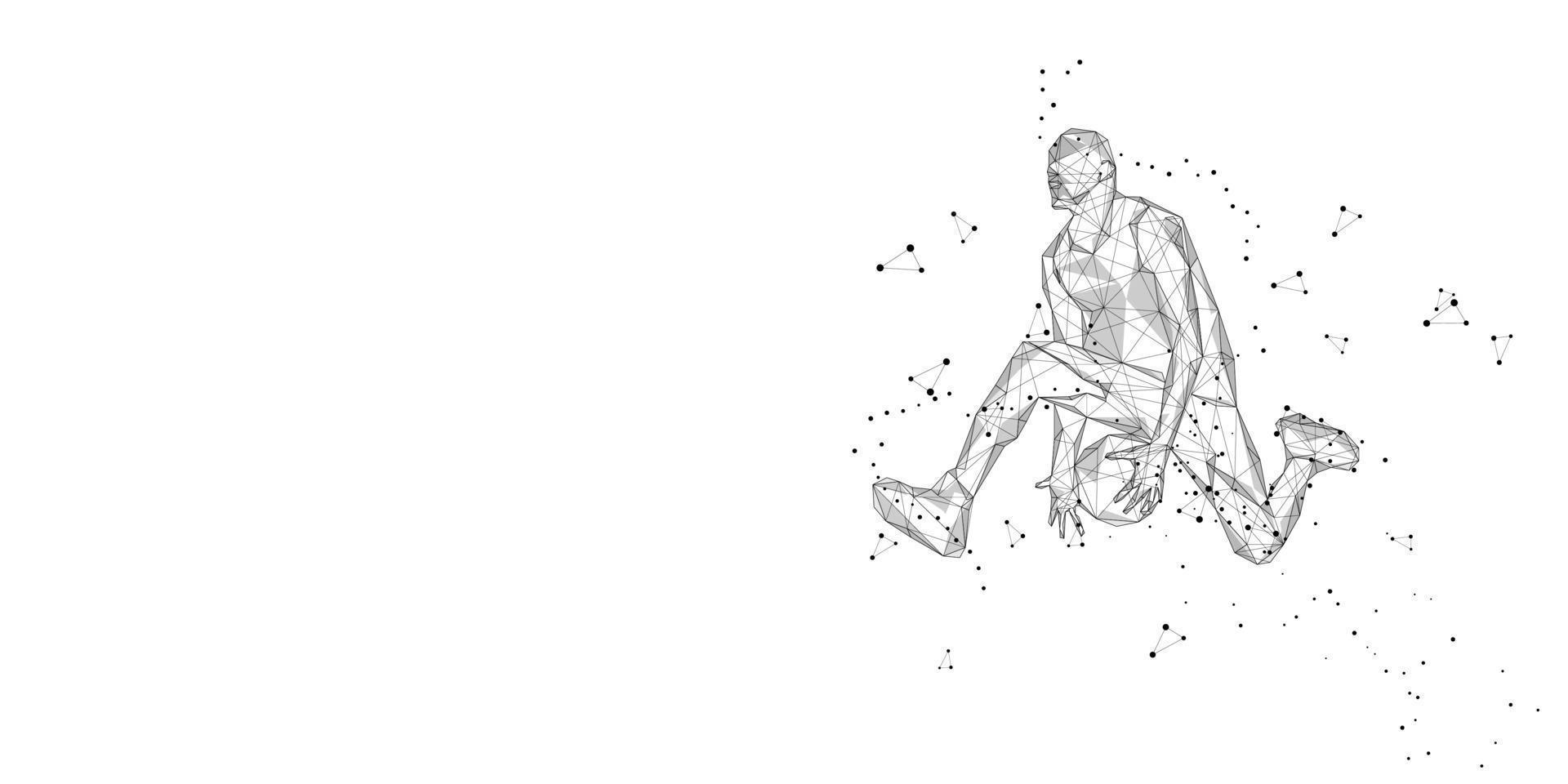The image is a meticulously detailed, black and white digital drawing, possibly computer-generated, featuring a human figure in mid-air, resembling a basketball player. The figure, composed entirely of geometric shapes, lines, and dots, showcases a complex network of interconnected coordinates. It appears to be passing a basketball from one hand to the other beneath its outstretched left leg, while the right leg extends behind it. The background is stark white, accentuating the intricate black and gray patterns that form the figure. Surrounding the protagonist are numerous black dots and lines, some forming small triangles, creating the illusion of constellations around the airborne figure.